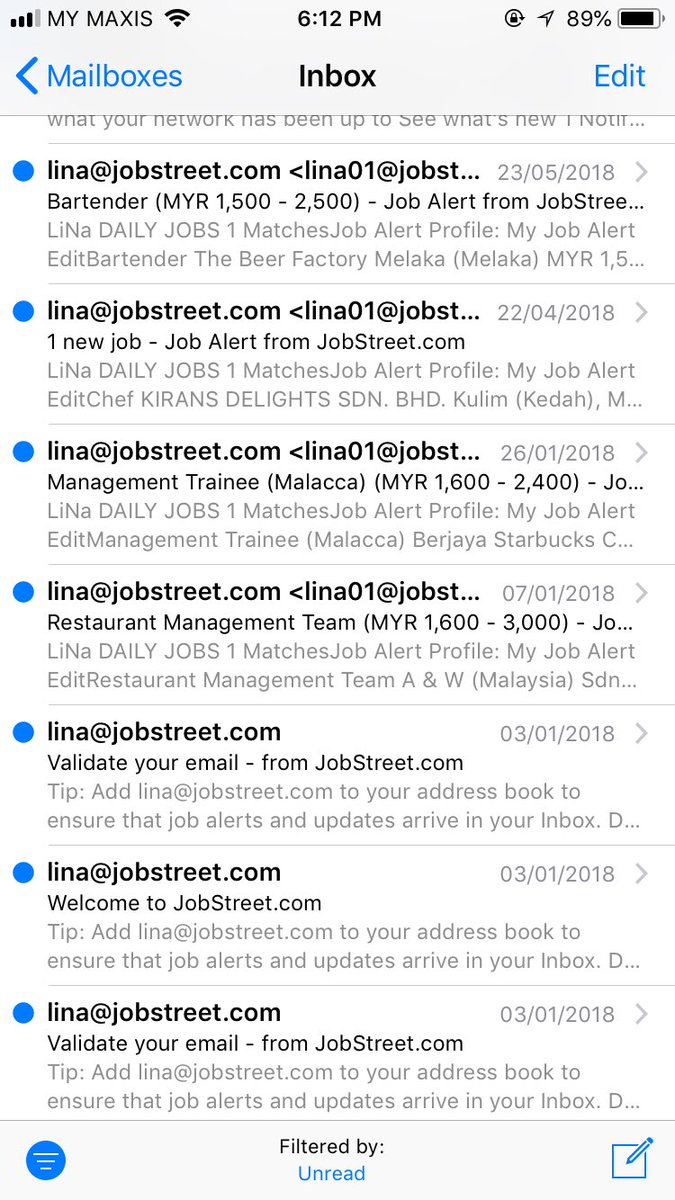This screenshot depicts the interface of an email account on a mobile device, captured at 6:12 PM. The upper section, approximately one and a half inches in height, features a light gray background. At the top left, there is a signal strength indicator displaying three or four black bars, signifying a strong Internet connection, followed by the label "MY MAXIS" in all capital letters. Adjacent to it is a fully-lit Wi-Fi icon.

Centered at the top is the current time, 6:12 PM, and to the right, the battery icon, which is predominantly black with a slight gray fill on the right side, indicates an 89% charge. Next to the battery icon are an arrow icon and an account icon, followed by a greater-than sign pointing to the left, indicating possible navigational controls.

Below this upper section, the interface transitions to a white background. In blue text, the left side reads "Mailboxes," the center displays "Inbox" in black, and the right side shows "Edit" in blue.

The list of emails begins immediately below, with each entry featuring a blue circle icon on the left. To the right of each circle is the sender's name, and further right is the date the email was sent. Each email entry comprises a headline followed by two lines of preview information. The first email's details are partially visible, showing a sender's name, "LINA" at jogstreet.com, followed by "LINA01 at jobstreet.com," repeated across seven entries.

At the bottom left corner, there's a blue circle encasing three white horizontal lines, likely indicating additional options or a menu. In the center bottom, "Filtered by" is written in black, with "Unread" in blue underneath it. Finally, in the bottom right corner is a square icon with a pencil protruding from its upper right corner, likely the compose button.